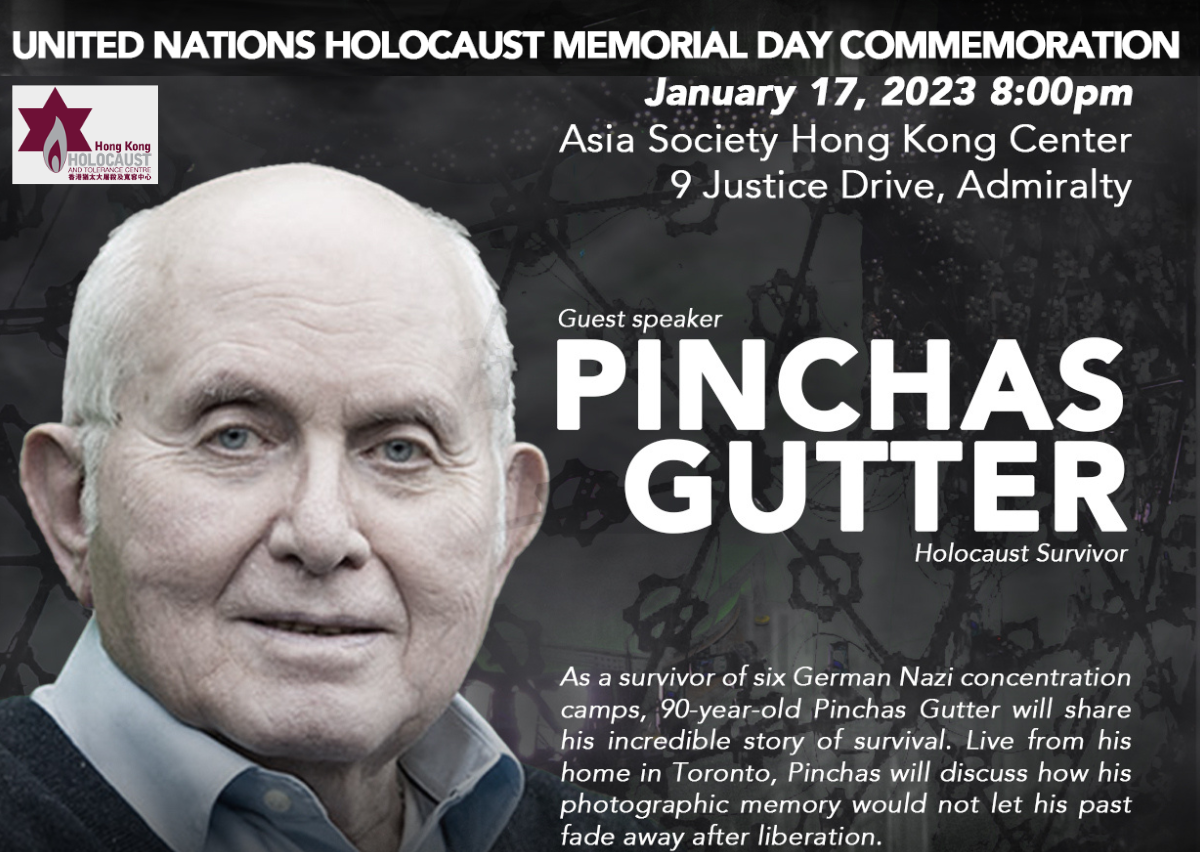The image is a black and white advertisement for the United Nations Holocaust Memorial Day Commemoration event. At the very top, in white print, it reads "United Nations Holocaust Memorial Day Commemoration," followed by the details "January 17, 2023, 8 p.m., Asia Society Hong Kong Center, 9 Justice Drive, Admiralty." In the upper left corner, there is a white square containing the logo of the Hong Kong Holocaust and Tolerance Center, featuring a red Star of David with a red and grey teardrop. Below the event details, on the left side of the image, there is a headshot of an older Caucasian man with blue eyes, bald on top with white hair on the sides, wearing a light blue button-up collared shirt. He is identified as the guest speaker, Pinchas Gutter, a Holocaust survivor, with text indicating that he survived six German Nazi concentration camps and will share his story of survival live from his home in Toronto, emphasizing his photographic memory and its role in preserving the past. The background of the advertisement is grey, with small circular images of flags present.